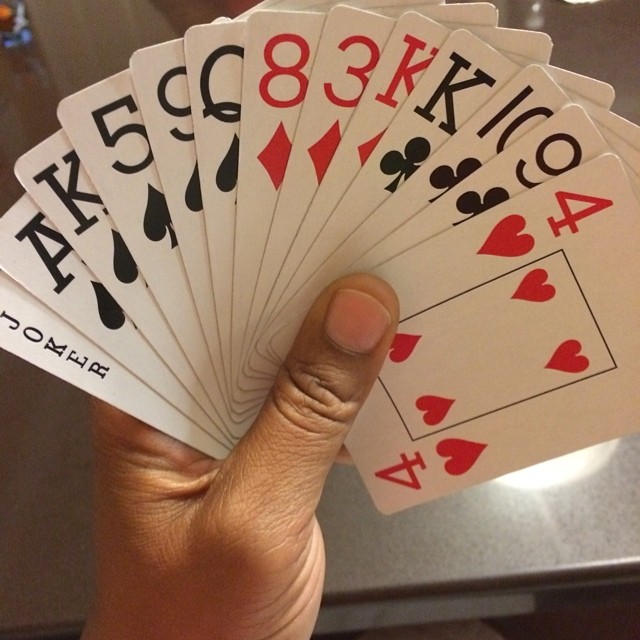A close-up photograph features a person holding a fanned-out deck of playing cards in their left hand. The image is sharply focused on the cards, with a minimalistic background dominated by a slightly reflective grey countertop. In the bottom right corner, the reflection of an overhead light adds a subtle detail to the scene. The deck is fanned out widely, showcasing a series of both black and red cards arranged sequentially from left to right. The visible cards include the Joker, Ace of Spades, King of Spades, Five of Spades, Nine of Spades, Queen of Spades, Eight of Diamonds, Three of Diamonds, King of Diamonds, King of Clubs, Ten of Clubs, Nine of Clubs, and finally, prominently displayed on the top right, the Four of Hearts. The red cards (Eight of Diamonds, Three of Diamonds, King of Diamonds, and Four of Hearts) stand out with their vivid coloration against the majority of black cards. The Four of Hearts is particularly noticeable, with its four red hearts framed by a black border, all set against a white background, symbolizing the balance and contrast within the deck.